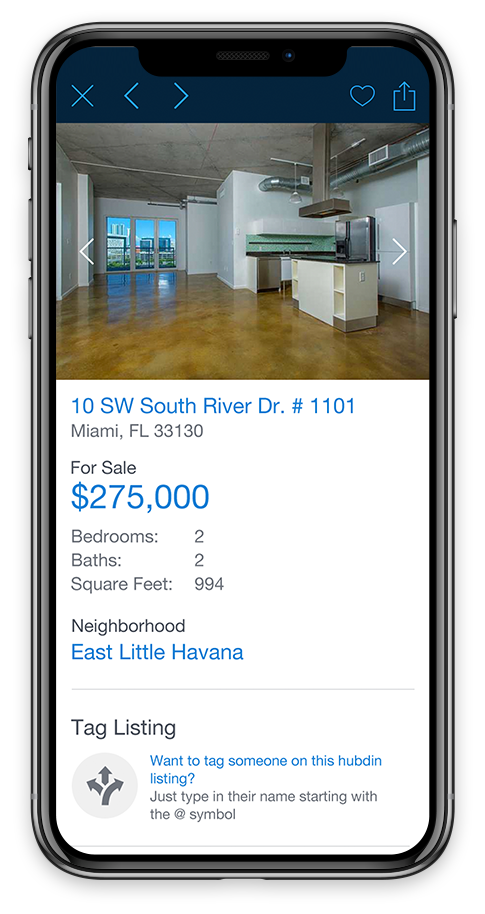The image displays the interface of a cell phone with a gray border. At the top, a dark blue bar features several light blue icons, starting from the left: an 'X', a left-pointing arrow, a right-pointing arrow, a heart, and a square with an upward arrow. The main image portrays the interior of a home with brown hardwood floors and a white kitchen island topped with black. A refrigerator stands against the back wall. At the far end, long windows or possibly a patio door reveal the outdoor sky and adjacent buildings. Below the image, blue text reads: "10 SW South River Drive, #1101, Miami, Florida 33130, for sale $275,000." Information beneath this includes: "Bedrooms: 2, Baths: 2, Square Feet: 994, Neighborhood: East Little Havana." Below this, a tag listing is followed by a circular icon with three arrows inside.